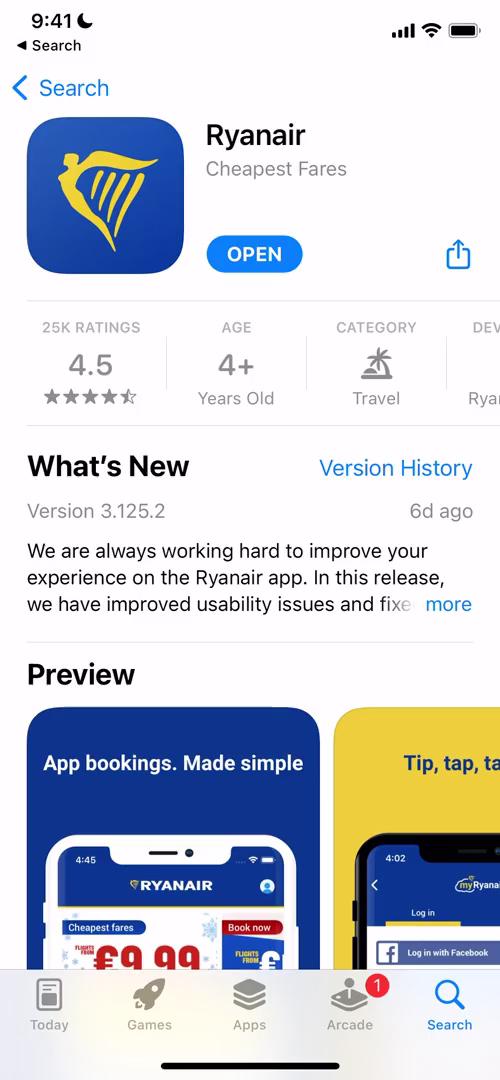The image displayed appears to be a screenshot from the Apple App Store, showcasing an app named "Rain Air." The interface features a clean, white background typical of the App Store. In the center, there is the blue and yellow icon for the Rain Air mobile application, which depicts an angel with strings resembling harp strings extending from its wings to its legs.

The listing highlights that the app is designed to help users find the cheapest airfares. Just below the app icon, there is a button labeled "Open," indicating that the app is already downloaded. The app boasts a rating of 4.5 stars from a substantial 25,000 users. It is rated appropriate for ages 4 and up and falls under the "Travel" category.

The description section mentions the latest update to version 3.125.2, released six days ago. The brief update note reads, "We are always working hard to improve your experience on the Rain Air app. In this release, we have improved usability issues and fixed..." The text trail ends with an option to read more.

Underneath the description, there is a preview segment showcasing the app's interface, accompanied by the tagline "App bookings made simple. Tap tap tap," with several illustrative images. Additionally, the bottom portion of the screen displays navigational buttons labeled "Today," "Games," "Apps," "Android," and "Search." The status bar at the top of the image shows standard icons for battery status, WiFi connection, and the current time, which reads 9:41, likely PM.